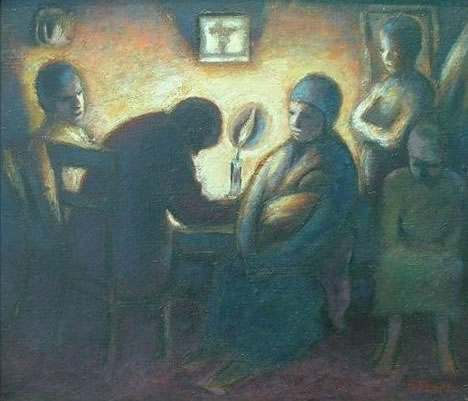The painting depicts a dimly lit, semi-abstract scene of five figures gathered around a table in a room bathed in the soft, golden glow of a single candle. The figures, some possibly men, women, and children, are rendered with rounded forms and pale, featureless faces, dressed in what appears to be old-style garments. To the left, one man sits mournfully with his head down, while a woman in a muted blue outfit with a head covering seems to be holding a baby. Another figure in a green dress sits near the bottom of the painting, faced by a standing figure with crossed arms. The room has a yellowish, marbleized wall, and the floor is a dark red. The background includes a picture frame and a hat—possibly a cowboy hat—hanging on the wall, completing the melancholic yet intimate atmosphere of the scene.